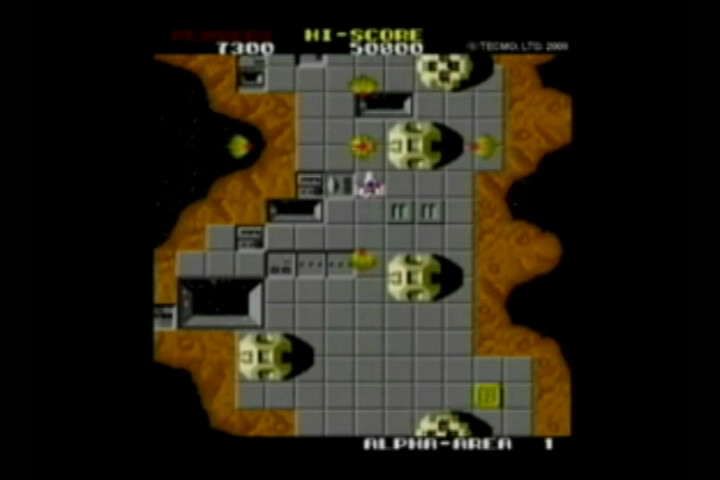In this top-down screenshot of a retro video game, the centrally positioned ground serves as a level that players must navigate. The scene features various obstacles blocking the apparent path, adding complexity to the terrain. At the top of the image, the current score of 7300 is displayed alongside the impressive all-time high score of 500,000. The bottom of the level is labeled "Alpha Arena 1," indicating the stage's name. The overall color scheme is relatively muted, dominated by grey for the floor, interspersed with patches of brown mud, and accentuated by dull green obstacles.